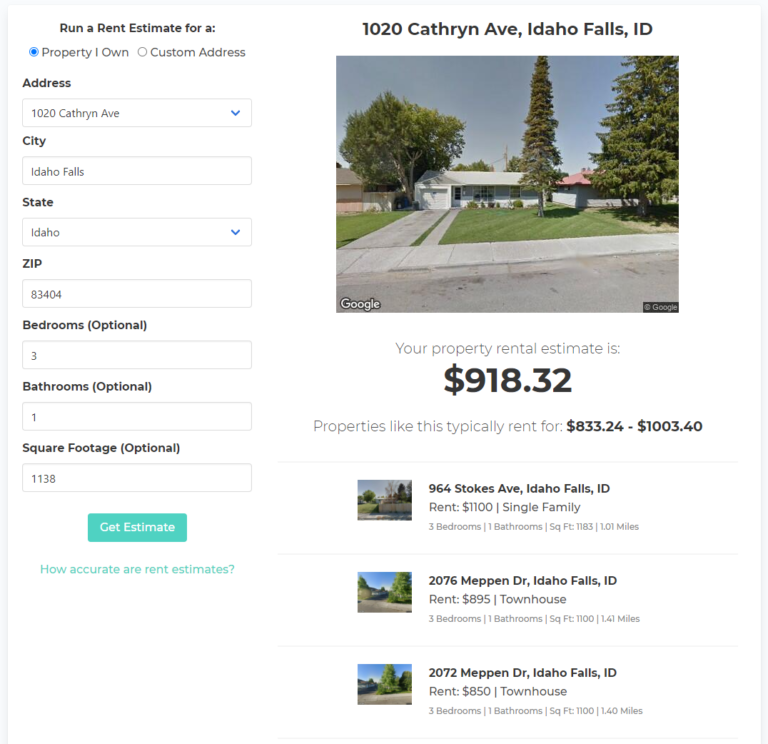Screenshot from a rental estimate tool (possibly Zillow) showcasing property details at 1020 Catherine Avenue, Idaho Falls, Idaho, 83404. The interface includes fields where users can input property information. For this address, the city is Idaho Falls, the state is Idaho, and the zip code is 83404. Additional fields include optional details like bedrooms (3), bathrooms (1), and square footage (1183 sq ft). A "Get Estimate" button allows users to receive an estimated rental value.

On the right side, 1020 Catherine Avenue, Idaho Falls, Idaho, is displayed prominently, accompanied by an image of the property. The house is a single-story structure with a one-car garage, a well-maintained lawn featuring an evergreen tree, and neighboring trees. The lawn is neatly cut, displaying visible mowing stripes. A green-grey label reads "Your Property," followed by a rental estimate of $918.32. The tool suggests that similar properties typically rent for between $833.24 and $1033.40. Examples of comparable rental prices in the area are highlighted: $1100, $895, and $850.